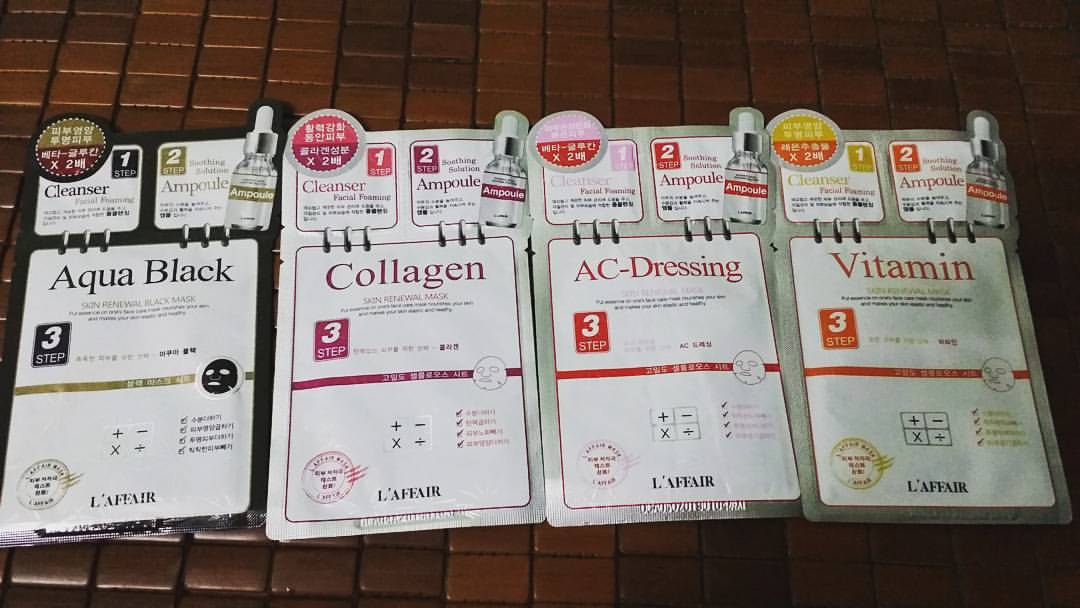The photograph showcases four sealed packets of skincare face masks laid out on a dark brown, tiled tabletop. Each packet displays a sample image of its respective product and is labeled with its name in large, colored text accompanied by an eyedropper bottle icon denoting the product type. From left to right, the packets are: Aqua Black, a skin renewal black mask with a predominantly white design on a black background; Collagen, which features purple accents; AC Dressing, highlighted with red elements; and Vitamin, accented in orange. The packaging is bilingual, incorporating both French ("La Faire") and possibly Asian script (Chinese or Korean), indicating a blend of international branding. Each packet is designed for a two-step application process involving an ampoule, hinting at an intricate skincare regimen.